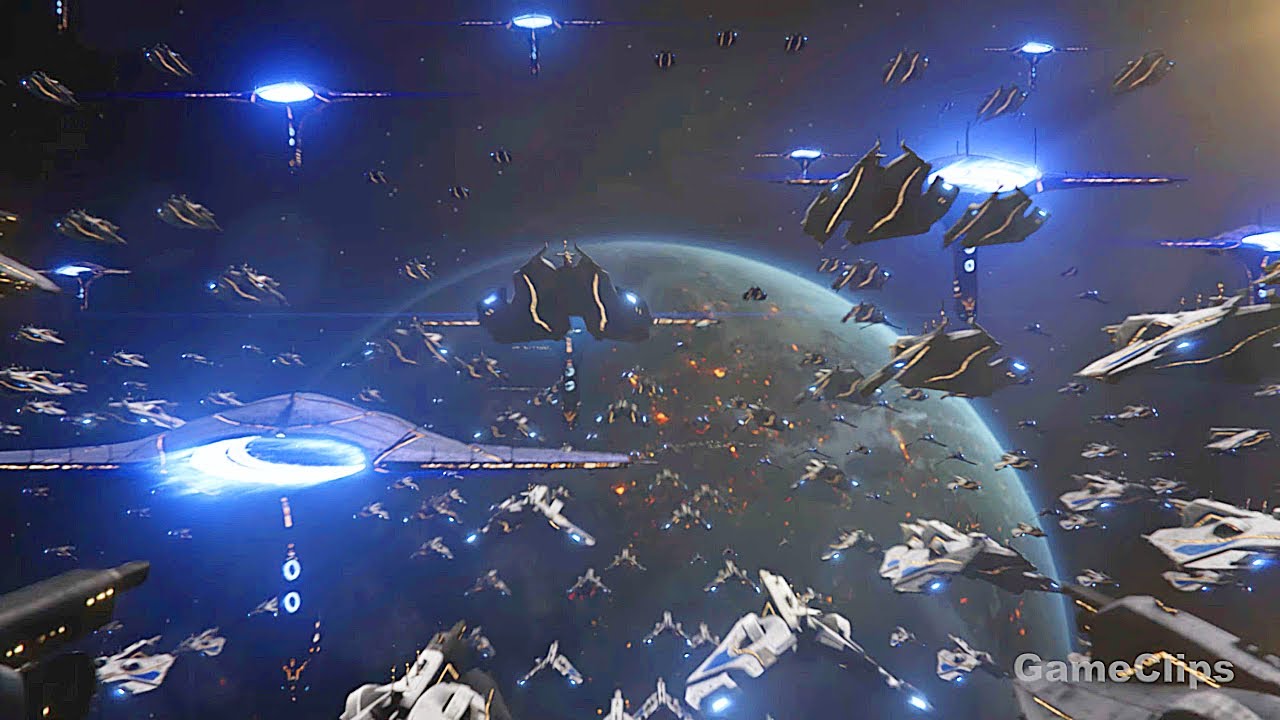This image appears to be an in-game screenshot from a sci-fi video game, featuring a fleet of futuristic spaceships flying in space. The ships, primarily black with yellow lines, and some white and gray, are equipped with blue energy trails streaming out of their engines, indicating they are traveling at high speeds. The background is a vast dark sky, characteristic of outer space. A large, glowing planet, possibly Earth, with significant blue and green coloration, is positioned in the distance, seemingly the destination for these hundreds of v-shaped spaceships. They appear to be moving in coordinated formations towards this planet, suggesting either an impending attack or a strategic maneuver. The bottom-right corner of the image bears the label "Game Clips," confirming its origin as a video game screenshot.